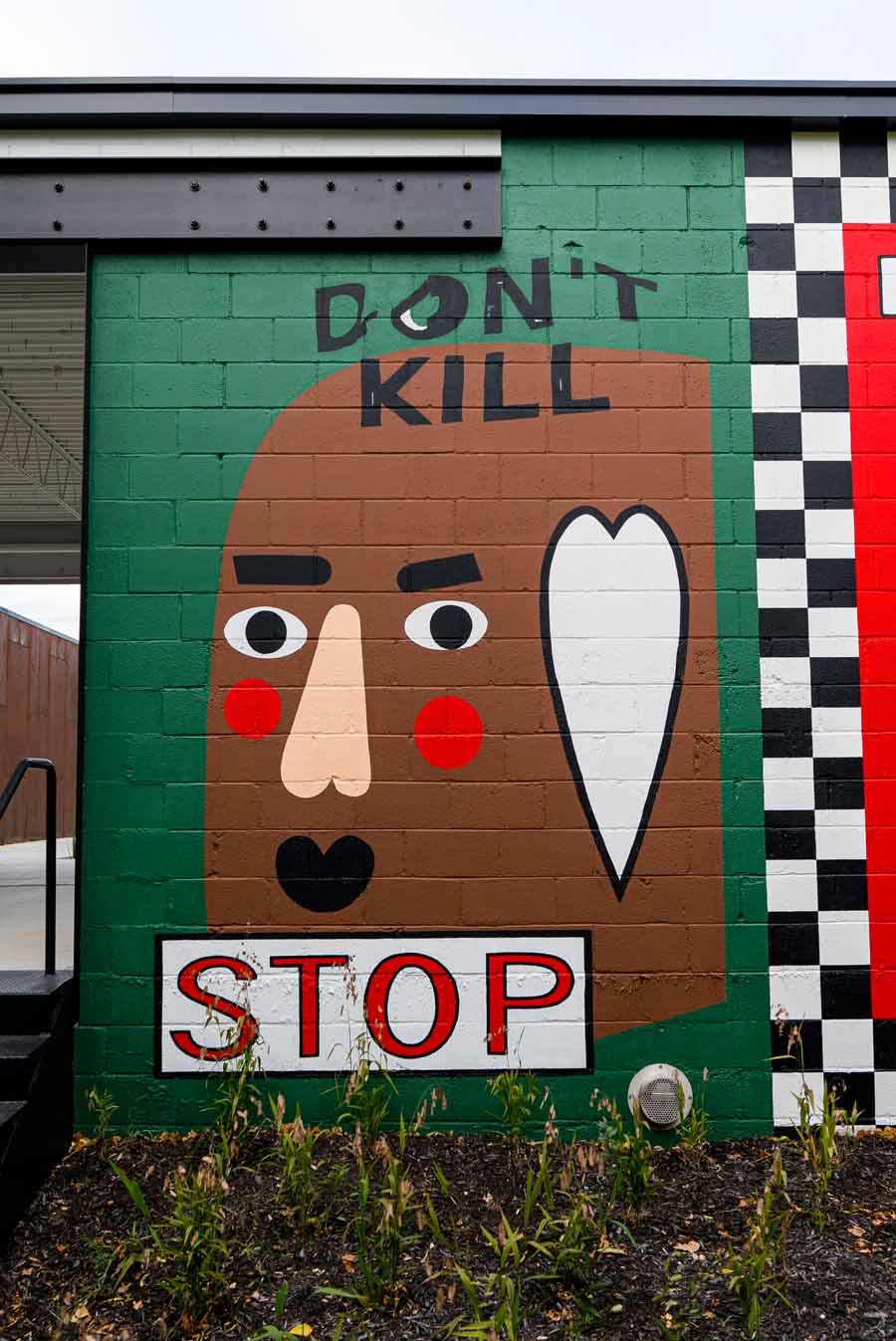The image showcases a vibrant and detailed mural painted on the side of a building's concrete wall, which is primarily painted in dark green. To the left of the mural, there is a set of black steps with a matching black railing, leading to a covered opening in the building. The right-hand side of the wall features a striking black and white checkered pattern, with some blocks distinctly painted in red.

Central to the mural is a brown figure that resembles a Mr. Potato Head, complete with individualized facial features including dark eyes, dark eyebrows, a beige nose, black lips, and red cheeks. A unique heart-shaped ear adds to its playful appearance. Above the figure, in bold black text, are the words "Don't Kill." Below it, a white rectangle outlined in black contains the word "STOP" in prominent red letters.

In the foreground, black dirt is visible with a few isolated stalks of plants and some green bushes planted in a row, adding a touch of natural life to the scene. The detailed artwork and the message it conveys create a powerful visual statement on the building's wall.